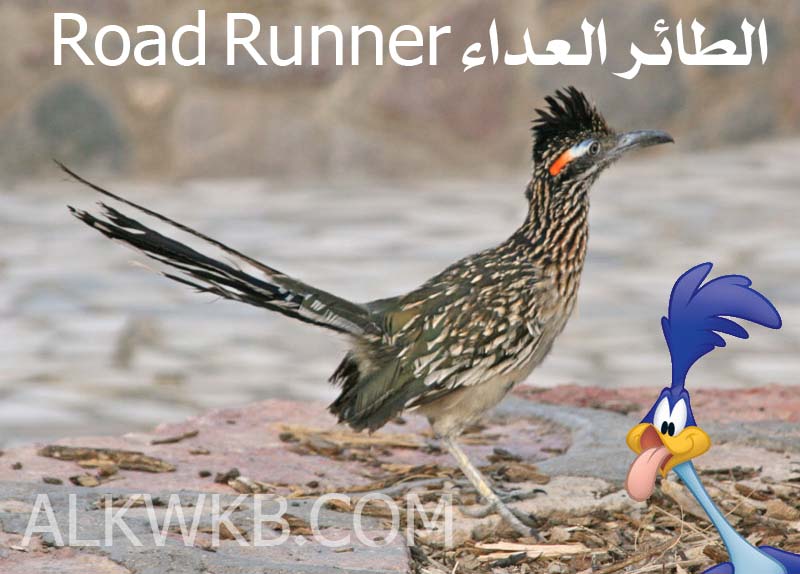The image is a detailed photograph of a roadrunner bird, centered and facing right, showcasing its distinctive profile. The bird boasts long, gray legs and a tail with darker feathers, protruding prominently. Its body features a beautiful mix of tan and gray feathers, complemented by a whitish underbelly. The bird's head is adorned with a striking black crown of feathers, resembling a mohawk, and it has an orange streak beside its eye. The beak is a dark gray, and an orangish-white-blue stripe is visible over its eye. Text at the top of the photograph reads "Roadrunner" in white sans serif font, followed by text in what appears to be Arabic. In the bottom left corner, there is semi-transparent text reading "ALKWKB.com." The bottom right corner features a blue cartoon version of the Looney Tunes Roadrunner, with a yellow beak, blue head feather, light blue body, visible wing tops, and a pink tongue sticking out. The overall setting appears to be outdoors, enhancing the natural allure of this fascinating bird.